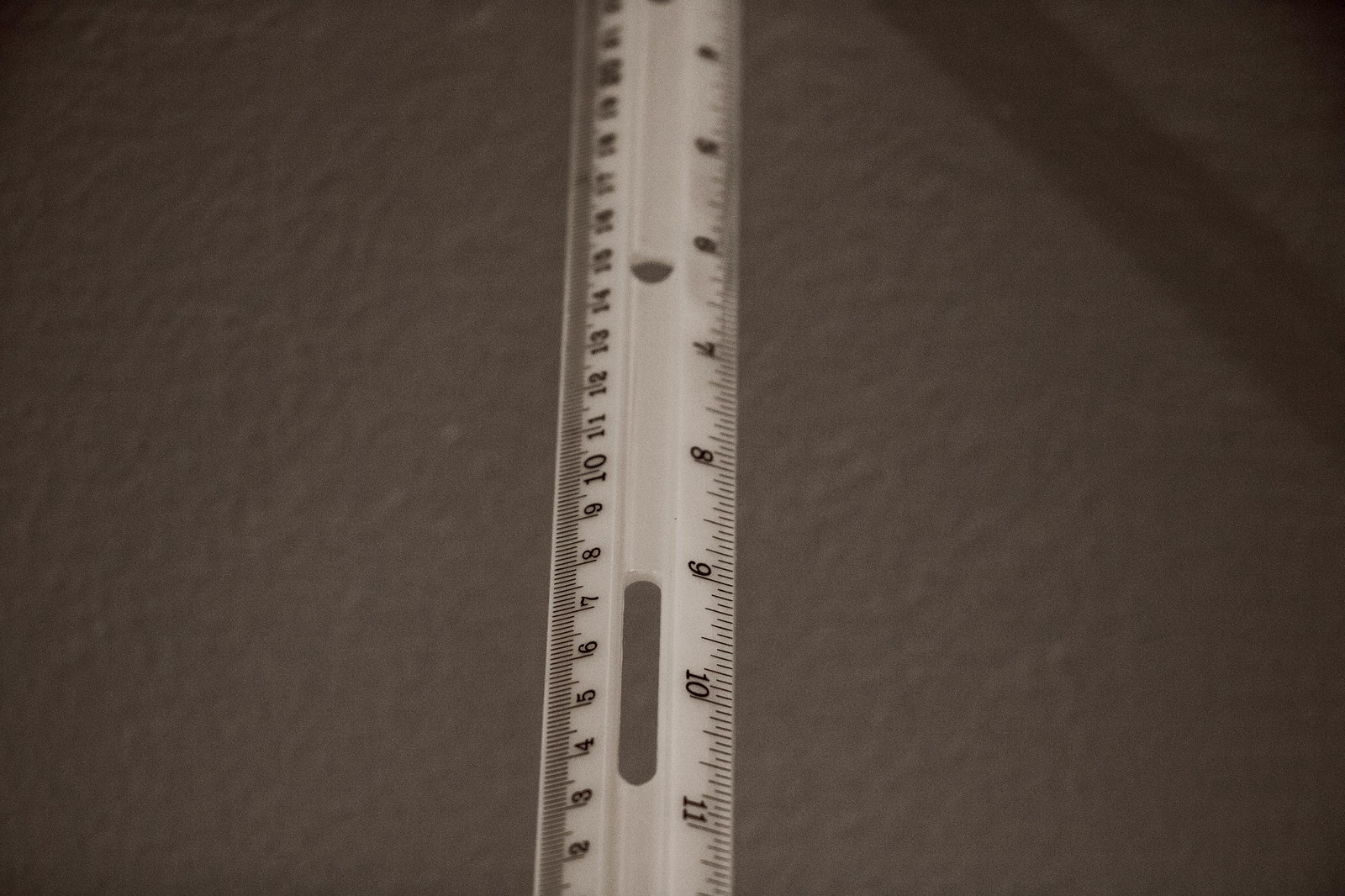The image features a white ruler positioned against a maroon background with a bumpy, wave-like texture. The ruler displays an inch scale on one side and a probable millimeter scale on the other. It is marked from just under 4 inches to slightly over 11 inches. The ruler has two notable holes: one in the center and another near its edge. The maroon surface appears textured for decoration, and a darker strip runs along the upper right corner, about an inch wide—possibly a shadow. The image focuses solely on the ruler against this uniquely textured backdrop.